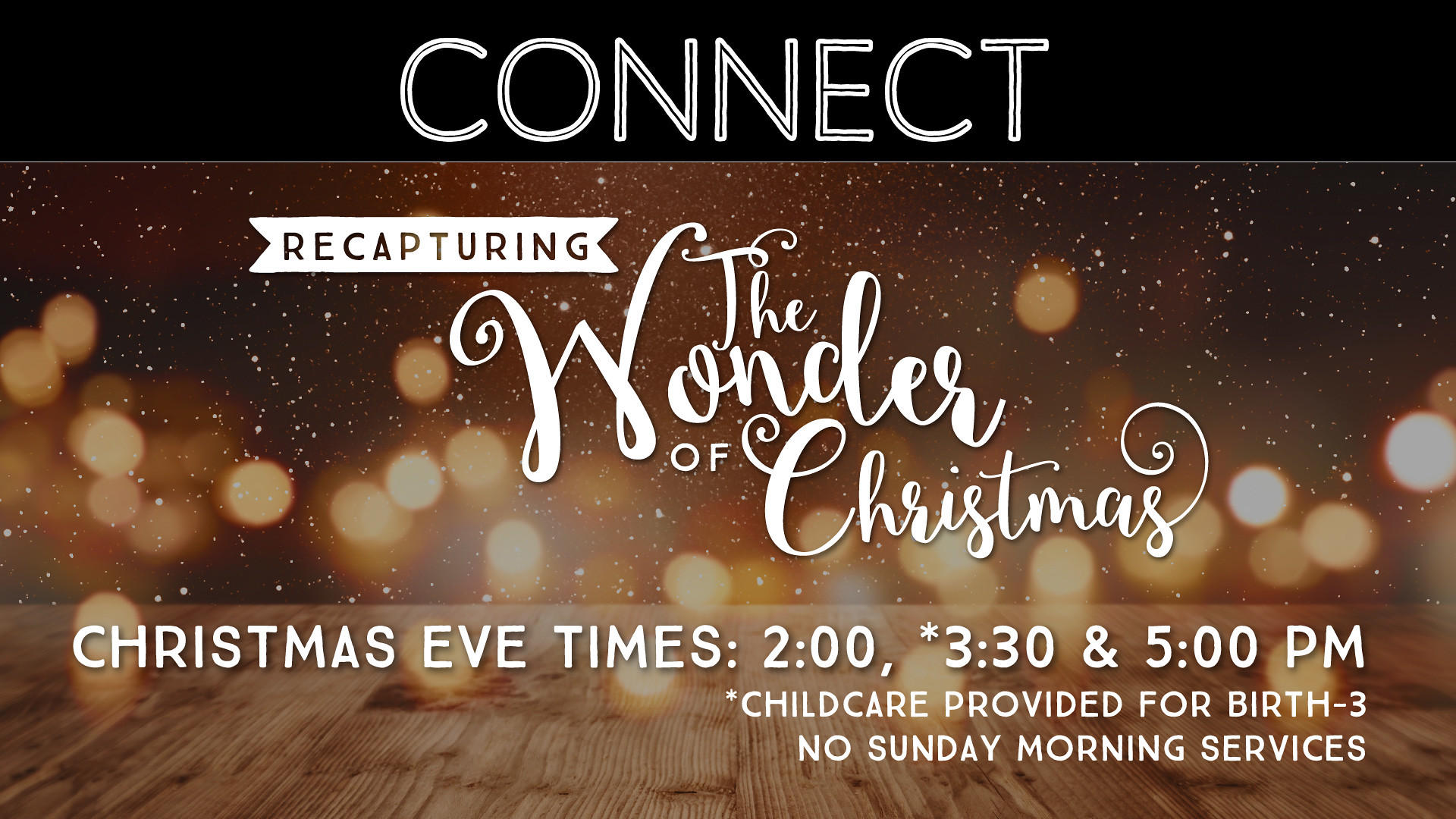The poster features a striking black bar at the top with the word "CONNECT" in bold white font. Below, a warm brown background adorned with twinkling white lights and scattered snowflakes sets a festive scene. Prominently displayed is a banner with the message "RECAPTURING THE WONDER OF CHRISTMAS," with "RECAPTURING" presented in negative space and "THE WONDER OF CHRISTMAS" elegantly scripted in cursive white letters. Further down, the poster lists "CHRISTMAS EVE TIMES: 2, 3:30, AND 5 P.M." in plain white block font. An asterisk notes that child care is provided for children from birth to three years old, followed by a reminder in white block text stating "NO SUNDAY MORNING SERVICES."